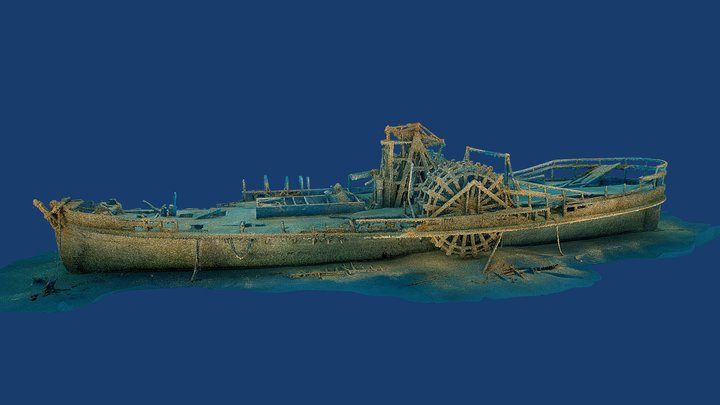The computer-rendered image depicts a shipwrecked vessel resting at the bottom of the ocean, enveloped in a deep blue background suggestive of underwater scenery. The ship, an intriguing blend of old and new design, features a rusted, elongated body partially buried in sand and debris, with the middle section more submerged than the front and rear, which protrude from the sandy ocean floor. Notably, a large, antique-looking paddle wheel is positioned on the side of the ship, reminiscent of a steamboat's propulsion system. The vessel exhibits signs of significant decay, including broken railings and scattered fragments around its sunken hull, emphasizing its aged and deteriorated state.